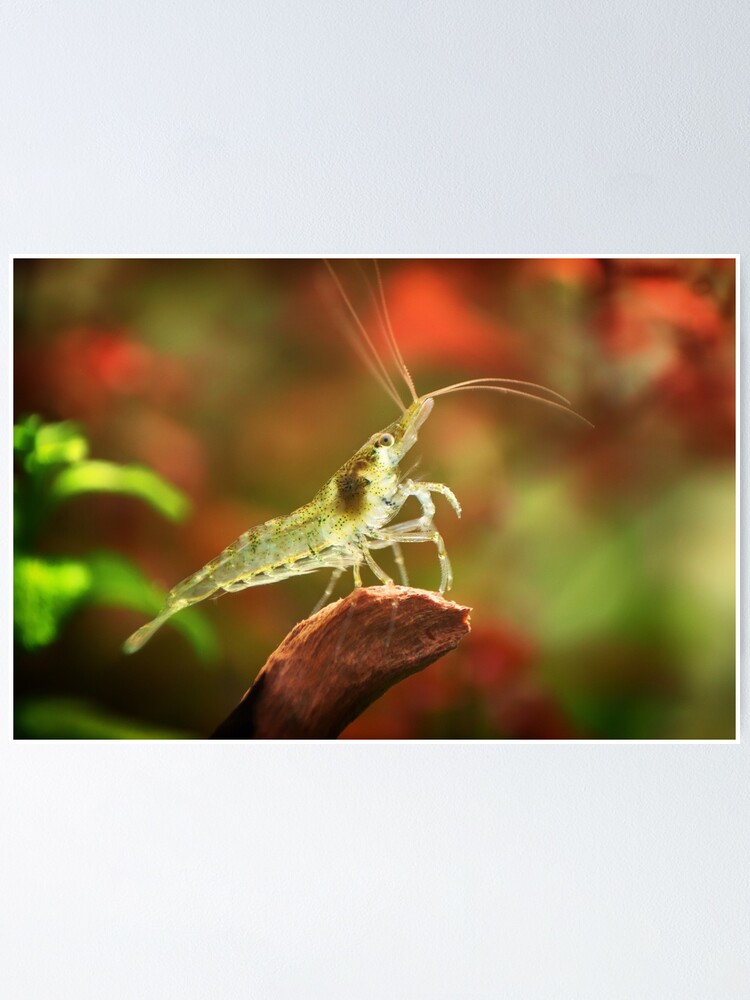Perched on a weathered piece of driftwood, a translucent crawfish, reminiscent of a miniature lobster, rests gracefully. The delicate creature is adorned with wisps of green algae, adding a natural embellishment to its glass-like exoskeleton. Its slender antennae are prominently visible, probing the surroundings. The background is an abstract blur of vivid reds and greens, possibly hinting at out-of-focus flowers and foliage, creating a soft and colorful backdrop. On the left side, green leaves emerge into the foreground, adding layers to the composition. The scene captures a moment of stillness before this clear, captivating crustacean potentially becomes part of a culinary journey.